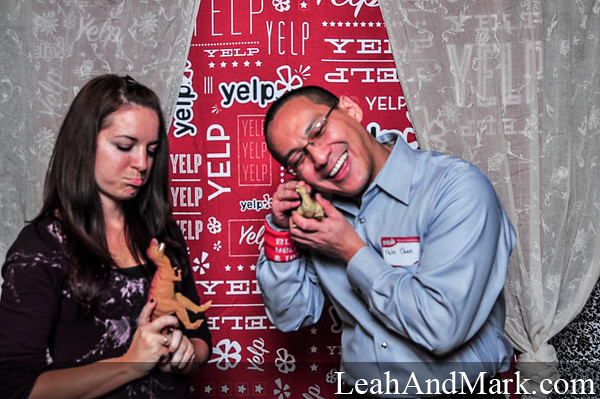In this vibrant and playful scene set against a stylish backdrop for a Yelp event, a man and a woman, likely in their early 30s, pose in front of a giant collage poster displaying varied fonts of the word "Yelp." Framing the picture are transparent white curtains with a subtle floral print, through which the bold Yelp logos are still visible. 

The woman, positioned on the left, sports a long-sleeve black shirt with intricate white detailing and has long, straight, shiny dark brown hair. She holds a tan Tyrannosaurus Rex action figure, her expression showing a pouty frown as she looks down at it with a touch of sadness.

To her right stands the man, exuding a contrasting cheerful demeanor. He wears a light blue button-up shirt, complete with a name tag on his right side and a red and white wristband, and has short black hair and glasses. With his head tilted and a joyous smile, he seems to be playfully interacting with his own smaller dinosaur figurine. At the bottom right corner of the image, the website "LEAHANDMARK.COM" is displayed in white letters, adding an official touch to this whimsically detailed photograph.